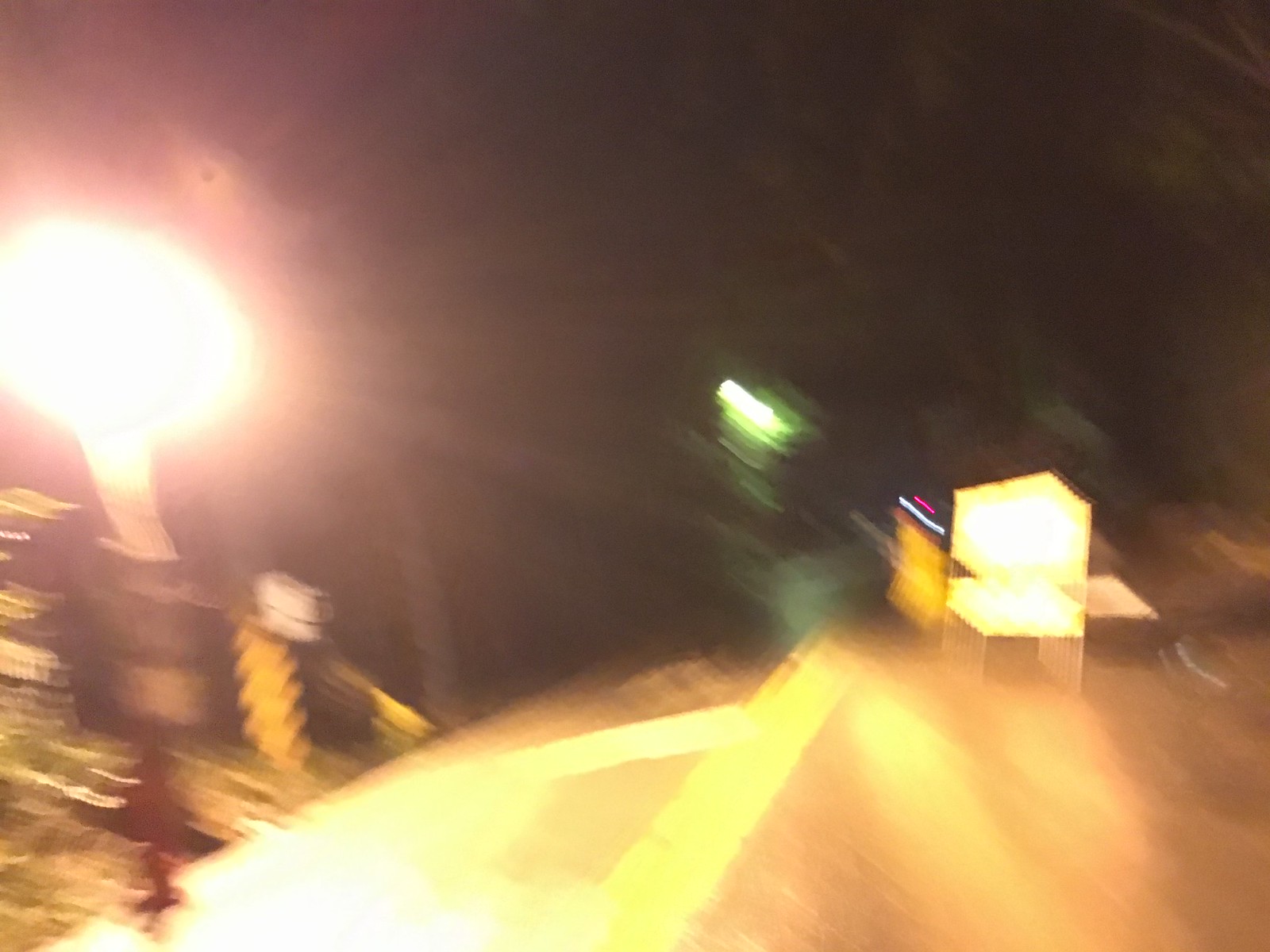To the left side of the image, there is a very bright light source. An indistinct object appears to be standing in the scene, partially illuminated by this intense light. In the far background, another light is visible, emitting a greenish glow that enhances the eerie atmosphere. The ground beneath showcases a stone texture interspersed with yellow lights scattered randomly. Further into the road, an object is subtly highlighted by yet another light, casting a notable glare across the scene. The overall composition suggests a night-time setting with various light sources creating a mysterious and almost surreal ambiance.